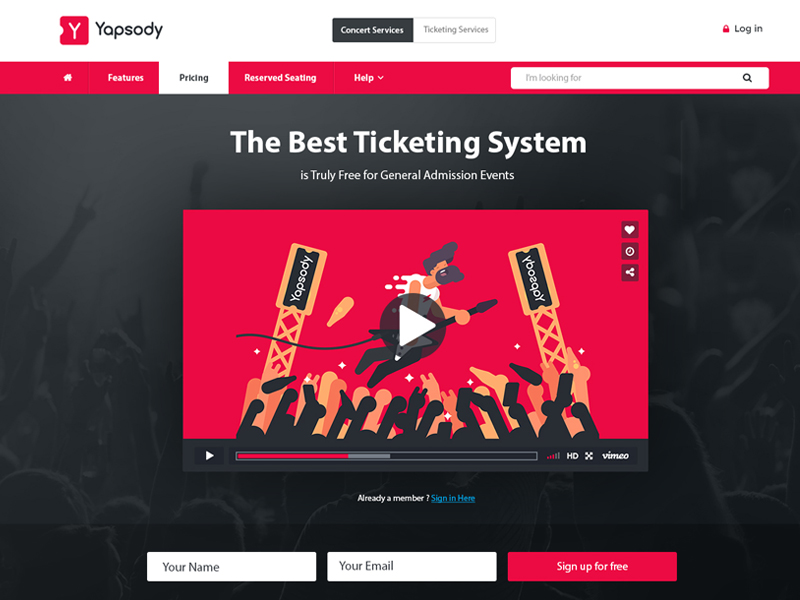This image is a screenshot taken from a website called Yapsody, which is a ticketing platform. The background of the webpage is predominantly black, adorned with vibrant red accents. The top of the page features the Yapsody icon, which resembles a red, square-shaped ticket with a white "Y" in the center.

Navigational elements at the top include icons and links for "Home," "Features," "Pricing," "Reserved Seating," and "Help." There is also a search bar with a magnifying glass icon labeled "I'm looking for."

The background image depicts a crowd of cheering silhouettes, arms raised, adding a dynamic atmosphere. In the foreground, a bold red rectangle contains the prominent white text "The Best Ticketing System," with smaller white text underneath proclaiming, "is truly free for general admission events."

Central to the image is a video player with a red background and a white play button. A progress bar shows that the video is about one-third played, indicated by a red line.

Below the video player are fields prompting the user to enter "Your Name" and "Your Email" to "Sign Up for Free."

This layout combines striking colors and clearly organized information, creating an engaging and user-friendly interface.